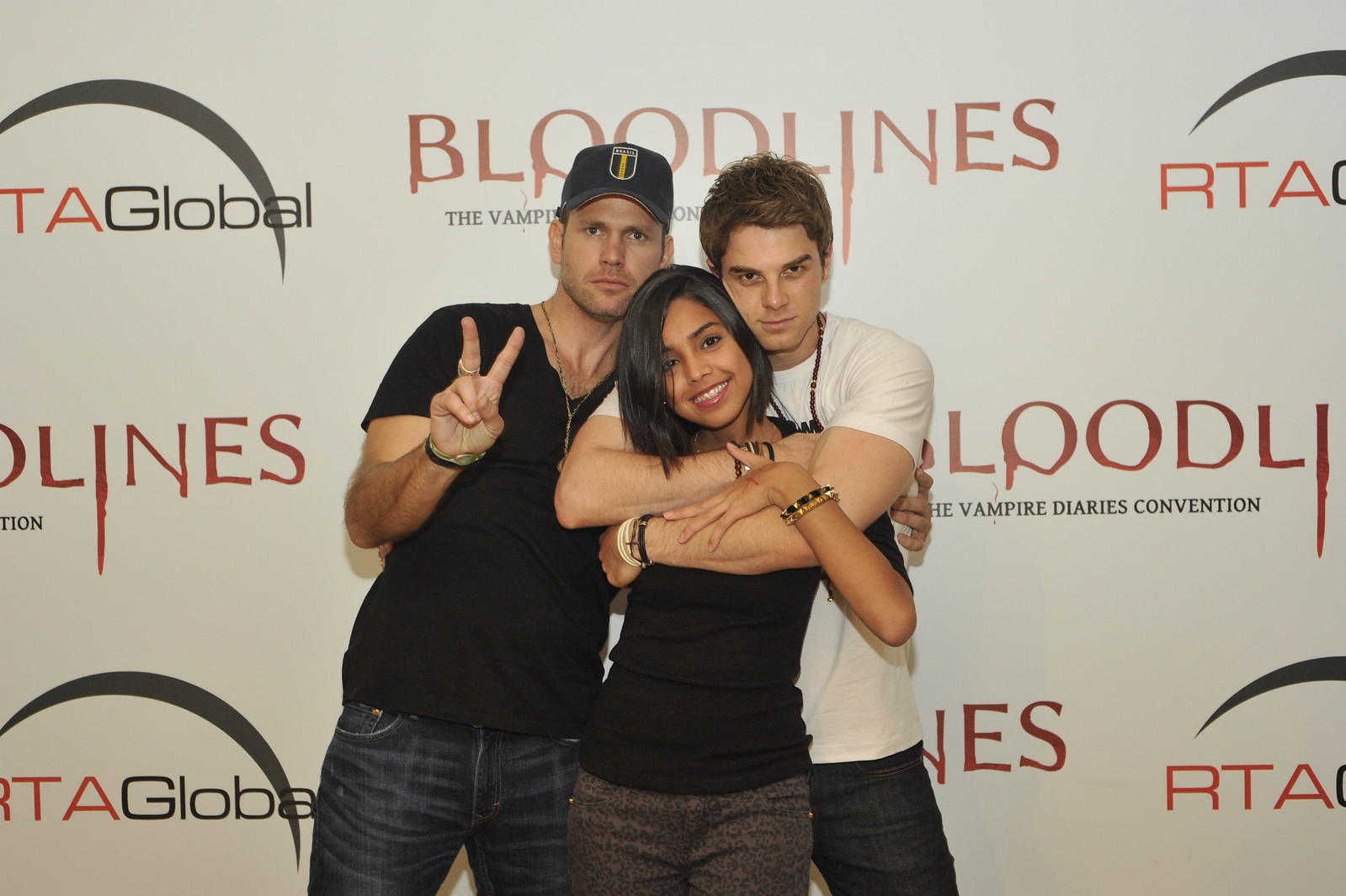In front of a white backdrop emblazoned with "Bloodlines, the Vampire Diaries Convention" and "RTA Global," three people pose for a photograph. The group centers around a young woman, who appears to be of Indian descent with straight, black, bob-length hair. She is smiling warmly, wearing a black shirt and gray pants. Behind her, the two men, identified as actors from the Vampire Diaries, stand with contrasting expressions. On the left, one actor is sporting a blue baseball cap with a logo, a black v-neck t-shirt, and dark blue jeans, and playfully holds up a peace sign with his right hand. On the right, the second actor, dressed in a white t-shirt and dark jeans, stands solemnly with his arms wrapped around the young woman in a protective embrace. His short hair complements his serious demeanor as he completes the tableau. The scene captures a heartfelt fan moment at the convention.